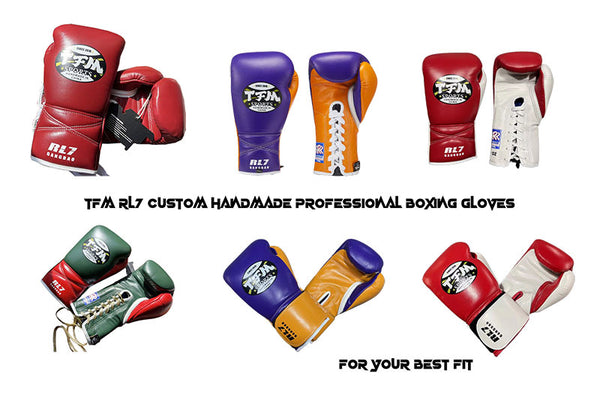The image presents a detailed advertisement for TFMRL7 Custom Handmade Professional Boxing Gloves, designed to offer the best fit. It features six pairs of high-quality boxing gloves, meticulously arranged in two rows of three. Each pair consists of one glove facing forward and the other facing backward to showcase both the front and back designs. The gloves prominently display the "TFM" logo on the padded area over the knuckles and include white laces for secure fitting.

On the top row, there are three distinctive color combinations: red and black, purple and yellow, and red and white. The bottom row mirrors a similar variety with green and red, another set of purple and yellow, and a final set of red and white. The model names and intricate stitching highlight the brand’s commitment to craftsmanship. The advertisement text, prominently centered between the rows, reads "TFMRL7 Custom Handmade Professional Boxing Gloves for your best fit," emphasizing both the product's quality and customization options. The image combines vibrant colors and professional presentation, making it ideal for use on websites or in magazines to effectively showcase the diverse range of gloves offered.